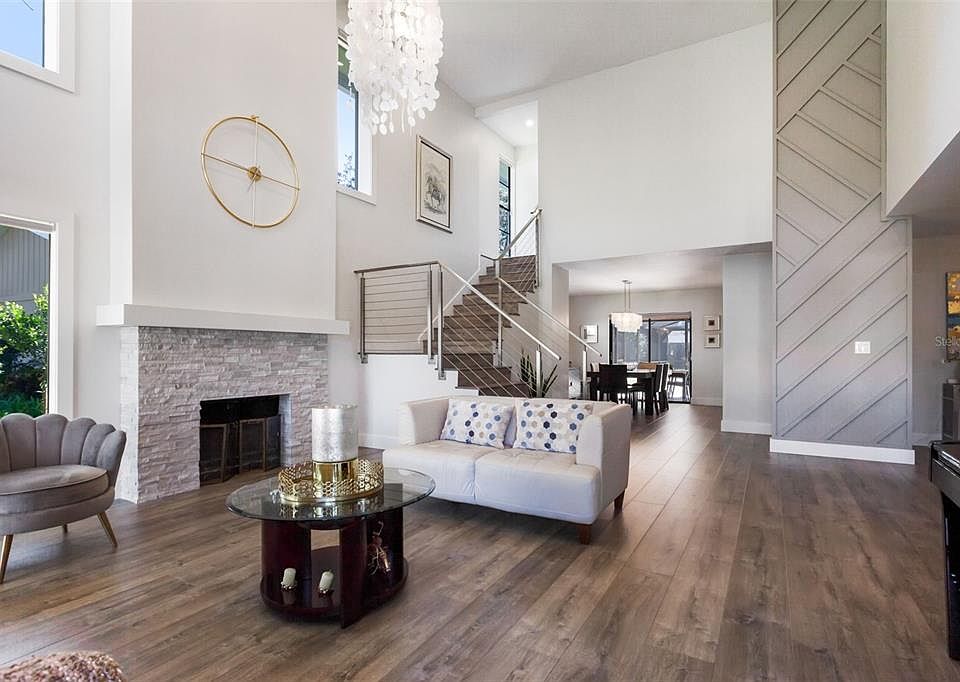This photograph captures the expansive and elegantly designed downstairs of a family home. In the foreground, a spacious living room boasts a high ceiling soaring up to the second story, approximately 20 to 24 feet tall. The open floor plan is accentuated by the rich, dark-colored wood flooring that seamlessly connects the various living spaces.

At the heart of the living room, near the fireplace, a white couch adorned with blue and white polka-dotted pillows faces a glass coffee table. Above the mantel, a striking golden clock with a circular design and cross in the center adds a touch of sophistication. The living room also features several seating areas, including modern chairs around a circular coffee table, providing ample space for relaxation and socializing.

A majestic crystal chandelier, described as both a chandelier and a collection of white shells, hangs prominently from the high ceiling, adding an opulent touch to the room. Near the living room, stairs lead up to the second story, hinting at additional spaces above.

In the background, the dining room is visible, highlighted by a crystal chandelier hanging above the dining table. A sliding door adjacent to the dining area opens up to the backyard, ensuring ample natural light floods the space. Overall, the thoughtfully designed interior, with its harmonious blend of elegant decor and functional spaces, exudes modern sophistication and comfort.